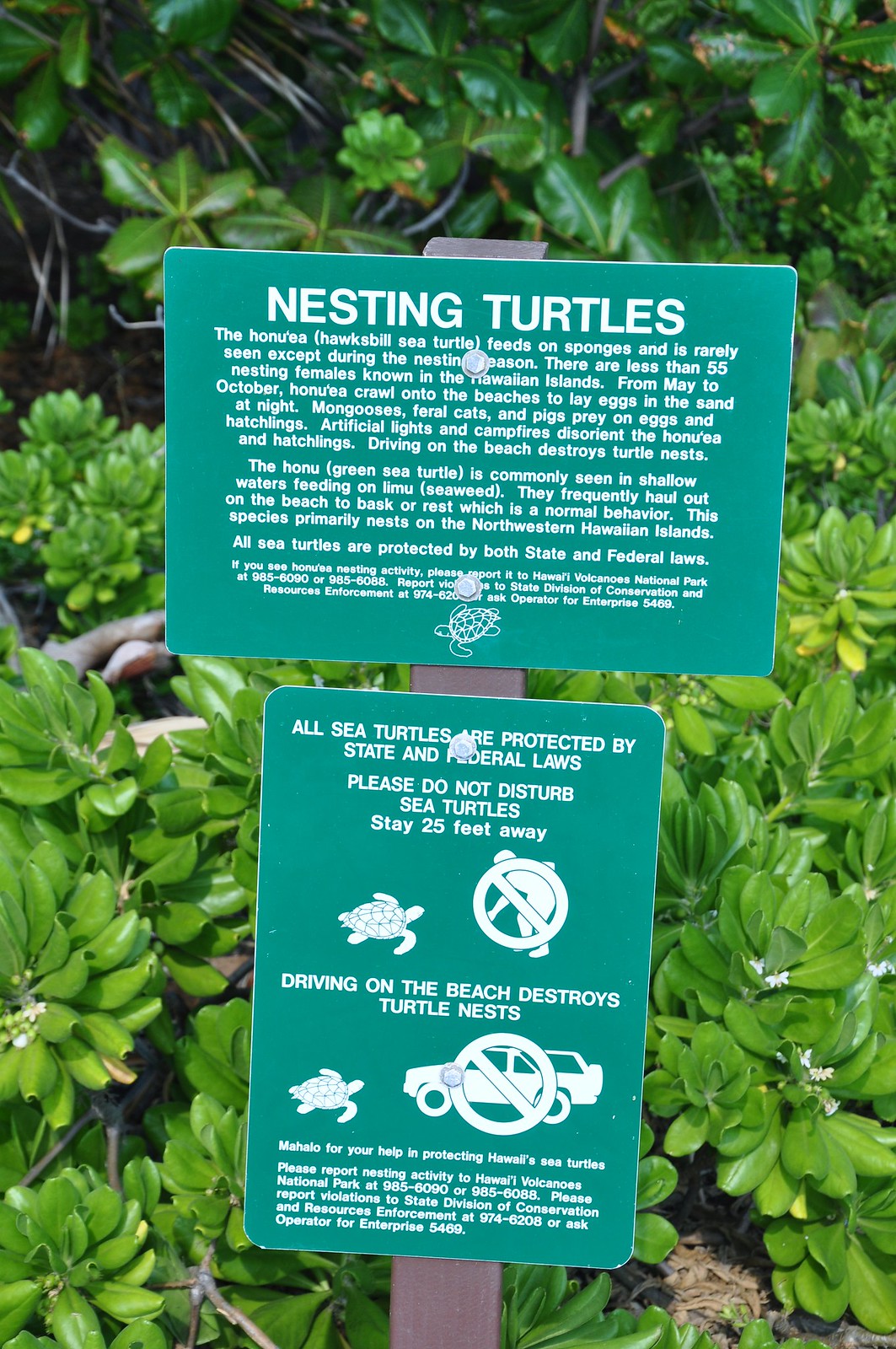In this tall, rectangular photograph taken in a lush, zoo-like area, two teal green, rectangular signs with white text are prominently displayed on a dark brown, grayish pole. The environment surrounding the signs features a vibrant array of bright, shiny green leaves, possibly palm leaves, set against a brown, mulch-like surface. 

The top sign, oriented horizontally, bears the title "Nesting Turtles" and includes several paragraphs providing detailed information about sea turtles, such as their nesting habits and the critical fact that there are less than 55 nesting females known in the Hawaiian Islands. Below this informational text is an image of a turtle.

The second sign, positioned vertically below the first, emphasizes the legal protections for sea turtles, stating, "All sea turtles are protected by state and federal laws. Please do not disturb sea turtles. Stay 25 feet away." This sign also features pictograms: one of a human bending down towards a turtle with a crossed-out circle indicating not to disturb the turtles, and another of a vehicle with a similar crossed-out circle warning against driving on turtle beaches, as it destroys turtle nests. This detailed description highlights the protective measures in place for these endangered creatures and the surrounding natural beauty.